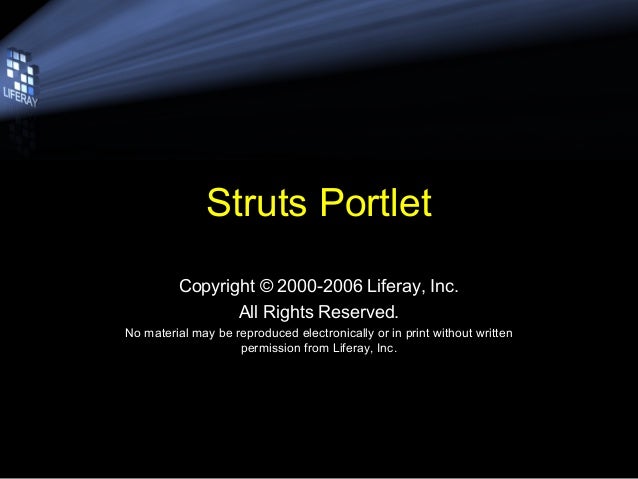The image depicts a digital slide with a predominantly black background. At the top, a stream of light in varying shades of blue creates a wave-like effect, extending from the upper left corner towards the right. In the upper left, there is a pixelated logo consisting of small blue squares forming a shape. The focal point is in the center, where yellow text reads "Struts Portlet." Below this, in white text, it states, "Copyright © 2000-2006 Liferay, Inc. All rights reserved. No material may be reproduced electronically or in print without written permission from Liferay, Inc." The slide features a combination of colors, including white, yellow, black, gray, blue, green, and tan, suggesting it might be part of a digital presentation or instruction manual.